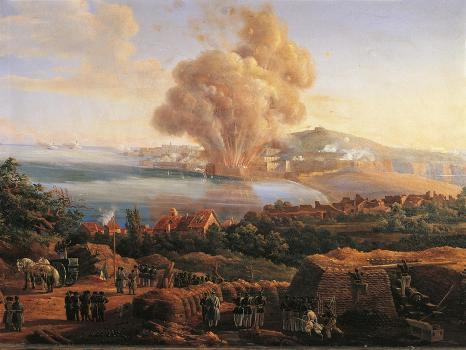The image is a detailed, wide canvas painting depicting a dramatic battlefield scene from the Revolutionary War in the United States. The foreground captures a battleground laden with orange-brown dirt and green trees, where soldiers in light-colored pants and dark tops stand behind a stone and sand fortification with a cannon. To the right, more soldiers are positioned near a brick structure with supplies. The left side of the foreground showcases a camp featuring horses, carriages, and another group of soldiers.

In the middle of the image, a significant explosion erupts near a fort, sending a sand-colored cloud into the blue sky. Below this chaotic scene lies a village composed of small houses by a bay, with a beach and the ocean extending to the left. There are also boats visible on the water, adding to the complexity and intensity of the setting. Toward the right side of the image, a mountaintop with a peak can be seen, enhancing the scenic backdrop of this historical battle depiction.